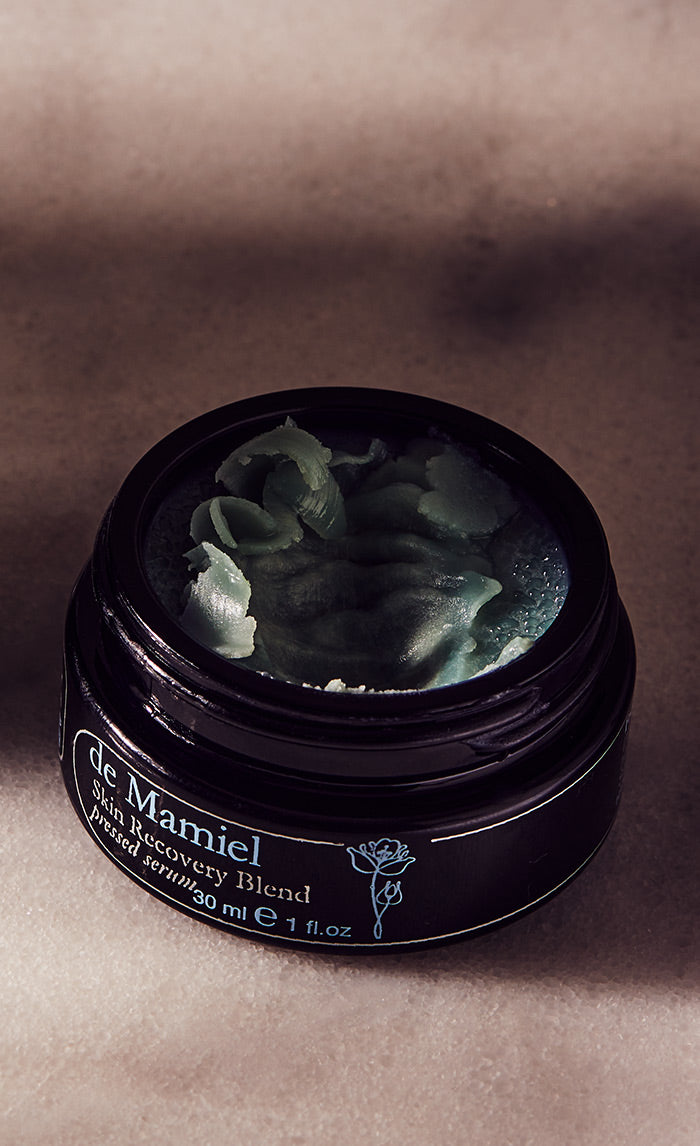The image displays an opened, small black jar containing a gel-like substance, which appears somewhat clear with dark undertones, possibly due to the lighting or angle of the shot. The label on the jar features a white border with the brand name "D. Mammiel" in light blue text, followed by the description "Skin Recovery Blend, Pressed Serum." It specifies the jar's contents as 30 mL (1 fluid ounce). The label also includes a design with two small flowers on the right side and a larger flower in the center. The jar’s contents have been disturbed, showing noticeable fingerprints where someone has scooped out the serum. The jar's surface indicates it's a dark, opaque material. The lid is missing, revealing the moist, salve-like texture inside, reminiscent of Vaseline, designed for application on skin areas in need of recovery or moisture.